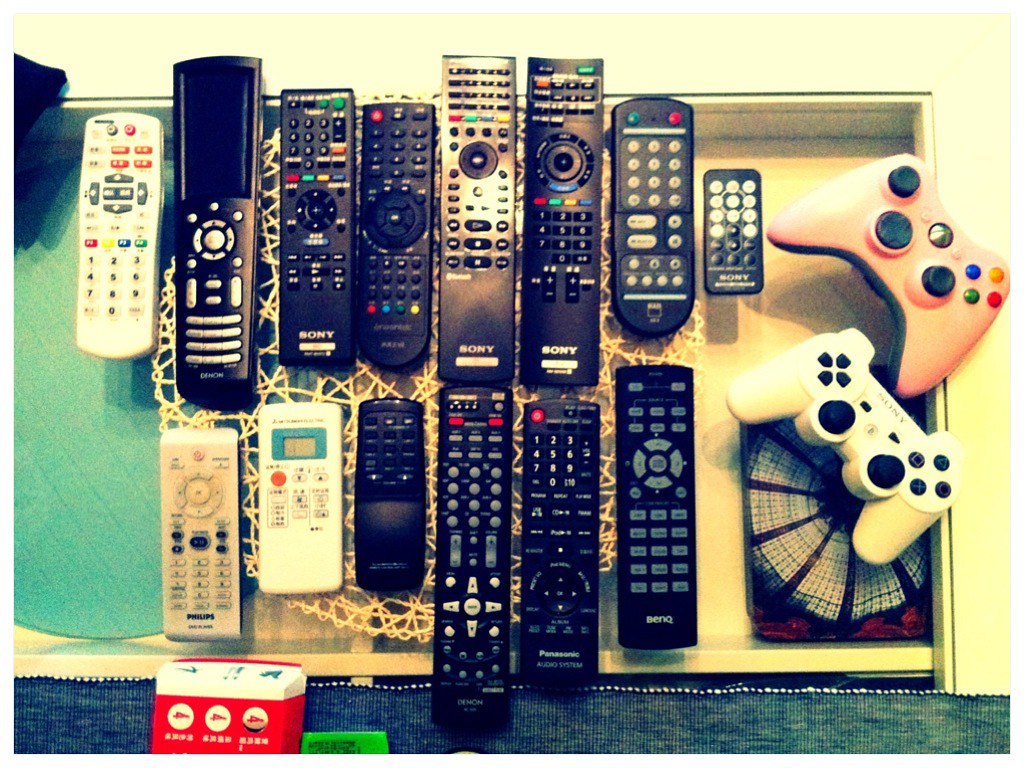In the slightly out-of-focus photograph, a white coffee table with a central glass panel houses a collection of decorative items, including teal and wicker doilies. Atop the table, arranged meticulously, are 14 remote controls of varying sizes and designs. While 11 of these remotes are black, three are white, each one distinct without any duplicates. Notably, on the bottom left, a red device and a neon green device are partly visible but extend out of frame. The right side of the table features a white Sony PlayStation 4 or higher controller and a baby pink Xbox controller. The table itself seems to rest on a yellow-framed drawer, with a green piece of fabric poking out from the left. Some remotes have colored buttons, including one with red arrow buttons at the top. The photograph also captures the eclectic mix of remote types, including TV remotes and console controllers, emphasizing the diversity and uniqueness of each device.